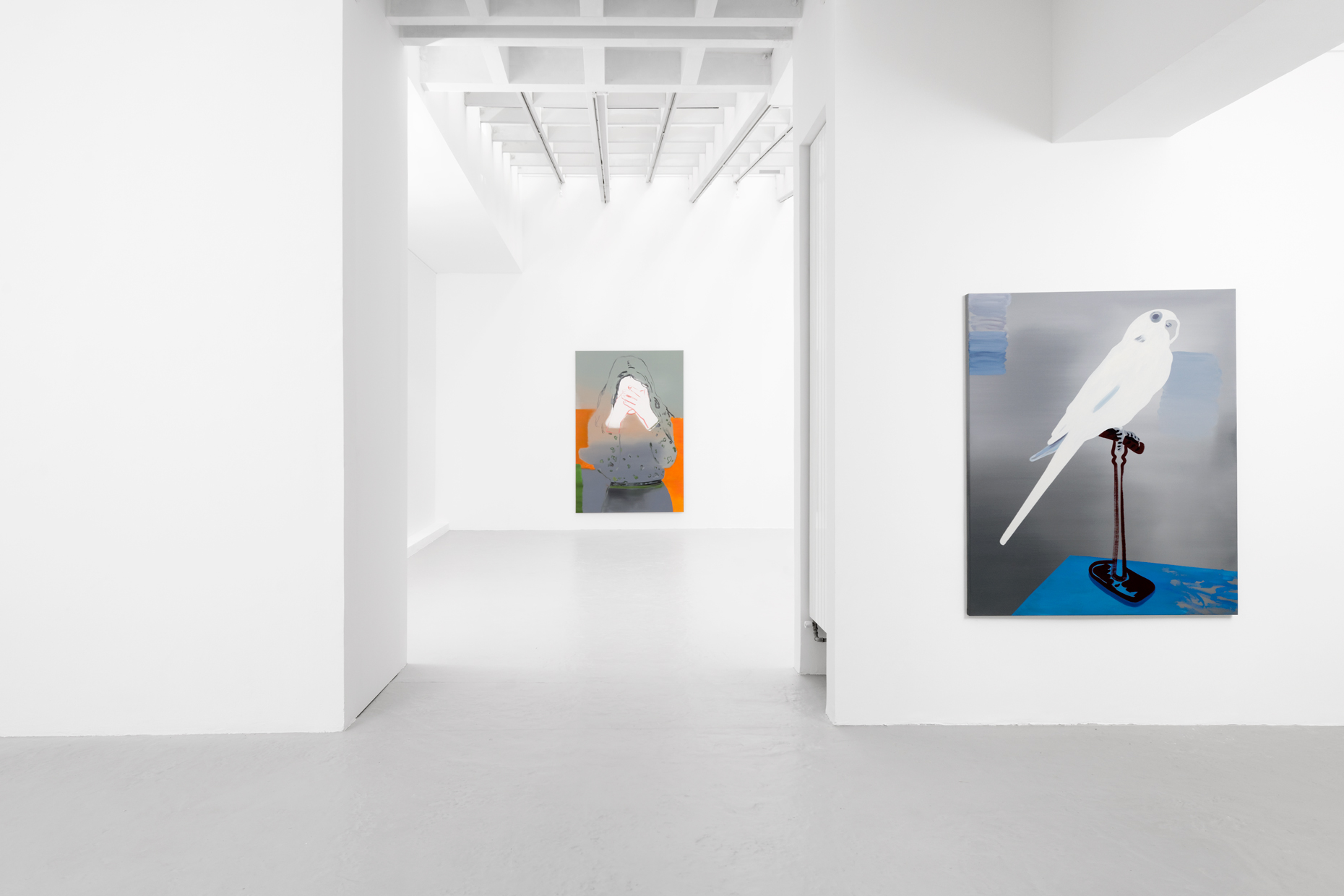The image showcases an art gallery with pristine white walls and a light gray floor, brightly illuminated by overhead lights. Central to the composition are two distinctive picture frames mounted on the wall. The first frame contains an image of a white parakeet perched on a short black bird stand with a crossbar at the top, set against a background that features shades of gray, white, and blue. Adjacent to it, in what appears to be an alcove, is a picture depicting a person with their head in their hands, dressed in hues of gray, white, dark gray, black, and orange, suggesting a contemplative or sorrowful mood. The room's minimalist design emphasizes the contrast and details of the artwork, contributing to a bright and clear ambiance with plenty of natural lighting, creating an inviting space for viewing these poignant pieces.